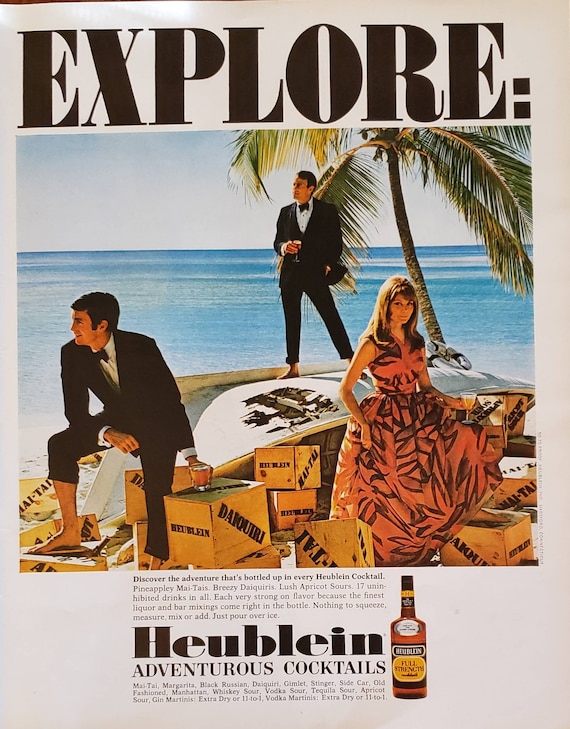In this vibrant magazine advertisement, the word "EXPLORE" is prominently displayed in bold, black capital letters at the top, inviting readers to delve into the world of Hubline's adventurous cocktails. At the bottom, the text introduces Hubline (spelled H-E-U-B-L-E-I-N) and encourages the discovery of the adventure encapsulated in every bottle. Central to the image, a suave gentleman, reminiscent of James Bond, stands confidently beneath a swaying palm tree. Beside him, a young woman exudes elegance in an eye-catching orange and black print dress. Adding to the exotic ambiance, another man, dressed in a tuxedo, has his pant legs casually rolled up to his knees, suggesting a leisurely stroll through the sand. The backdrop features a stunning ocean vista, with hues of blue and green blending seamlessly into the horizon, under a softly hazy sky. This scene captures the essence of tropical sophistication and the spirited allure of Hubline's cocktails.